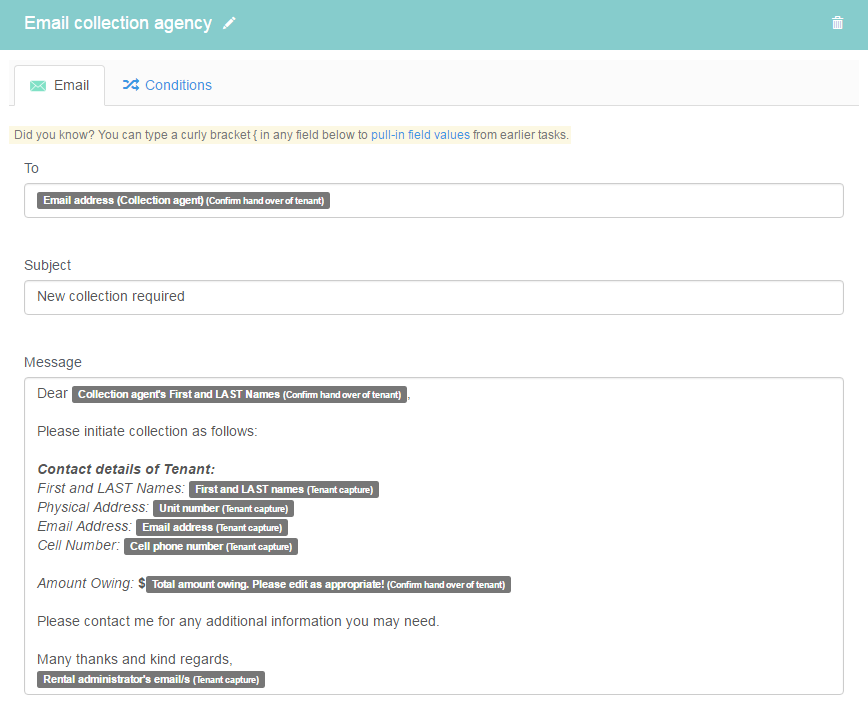The image depicts the interface of an email template creation tool, presumably part of a collection agency's system. The interface is primarily colored in tealish green and gray tones, providing a clean, professional look. 

At the top of the interface, there's a teal green bar with white text reading "Email Collection Agency" accompanied by a pencil icon for editing. On the far right of this bar is a trash can icon, indicating the option to delete.

Below this bar, there are two tabs. The left tab, labeled "Email," features a gray text with a lighter green envelope icon. Adjacent to it is the "Conditions" tab, marked by two crossing arrows and blue text.

The section below these tabs highlights a beige box with the text: 
"Did you know? You can type a curly bracket `{}` in any field below to pull in field values from earlier tasks." The phrase "pull in field values" is emphasized in blue.

Following this informational note, the template's content fields appear against a darker gray background. 

- **To:** A box labeled "Email Address (Collection Agent)" with additional context stating "Confirm Handover of Tenant."
- **Subject:** Another input box filled with the text "New Collection Required."

Underneath, the **Message** section begins with:
"Dear Collection Agent’s First and Last Names (Confirm Handover of Tenant)," where the term "Dear" appears distinct with appropriate spacing. 

The message continues in a structured format:
- "Please initiate collection as follows:"
- "Contact Details of Tenant":
  - "First and Last Names:"
  - "Physical Address: Unit Number"
  - "Email Address"
  - "Cell Phone Number"
- "Amount Owing: $Total Amount Owing"
- Closing remarks: "Please edit as appropriate! (Confirm Handover of Tenant)"
- Additional instructions: "Please contact me for any additional information you may need."
- Sign-off: "Many Thanks and Kind Regards,"
- Signature line: "Rental Administrators Email/s (Tenant Capture)"

These fields use varying font weights and colors to distinguish input areas and instructions, ensuring clarity and ease of use for the collection agent preparing the email template.